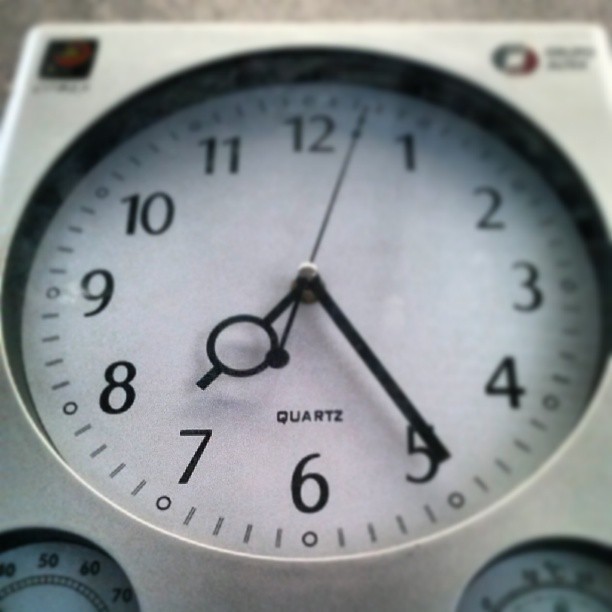This image showcases a square-framed clock with a round clock face nestled within the square. The clock features three distinct black hands: a shorter hour hand with a circular opening along its length, a longer and thicker minute hand, and a long, thin second hand. Branded by Quartz, this clock's design is both functional and aesthetically pleasing. Below the main clock face, two smaller round dials add detail and functionality to the overall design. The clock's intricate and precise mechanisms, coupled with its sophisticated appearance, exemplify Quartz's renowned craftsmanship.